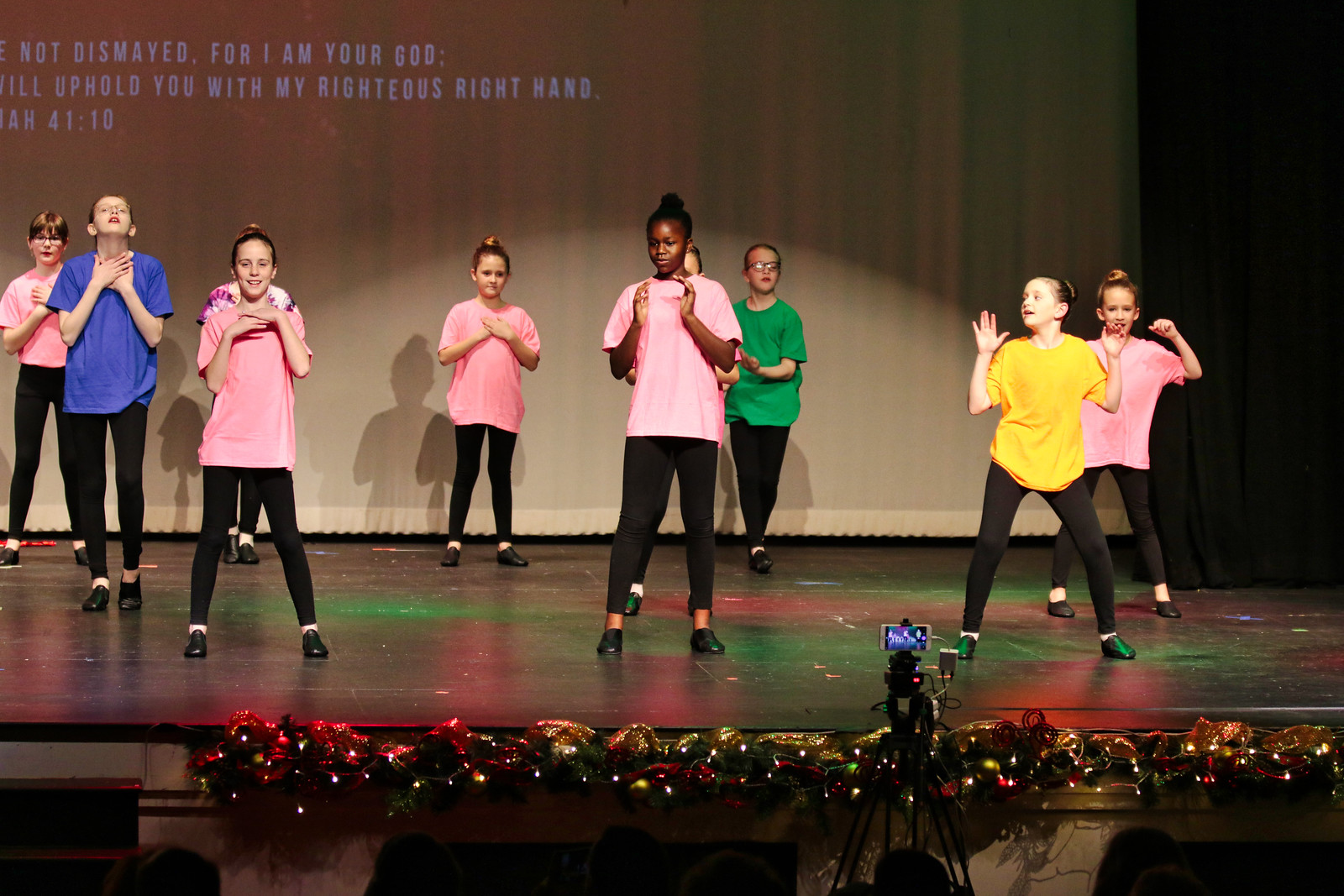In this image, a group of ten children, primarily girls and one African-American girl leading, aged approximately 10 to 14, are performing on a decorated stage adorned with tinsel and Christmas lights. They are all dressed similarly, wearing black pants and shoes. The majority are sporting pink shirts, while some are dressed in other vibrant colors like green, blue, and yellow. The backdrop features a screen displaying a Bible quote from Isaiah 41:10, "Do not be dismayed, for I am your God. I will uphold you with my righteous right hand." The children appear to be enthusiastically singing and gesturing, creating a festive and joyous atmosphere indicative of a holiday-themed religious performance. A camera is positioned to capture their lively presentation.